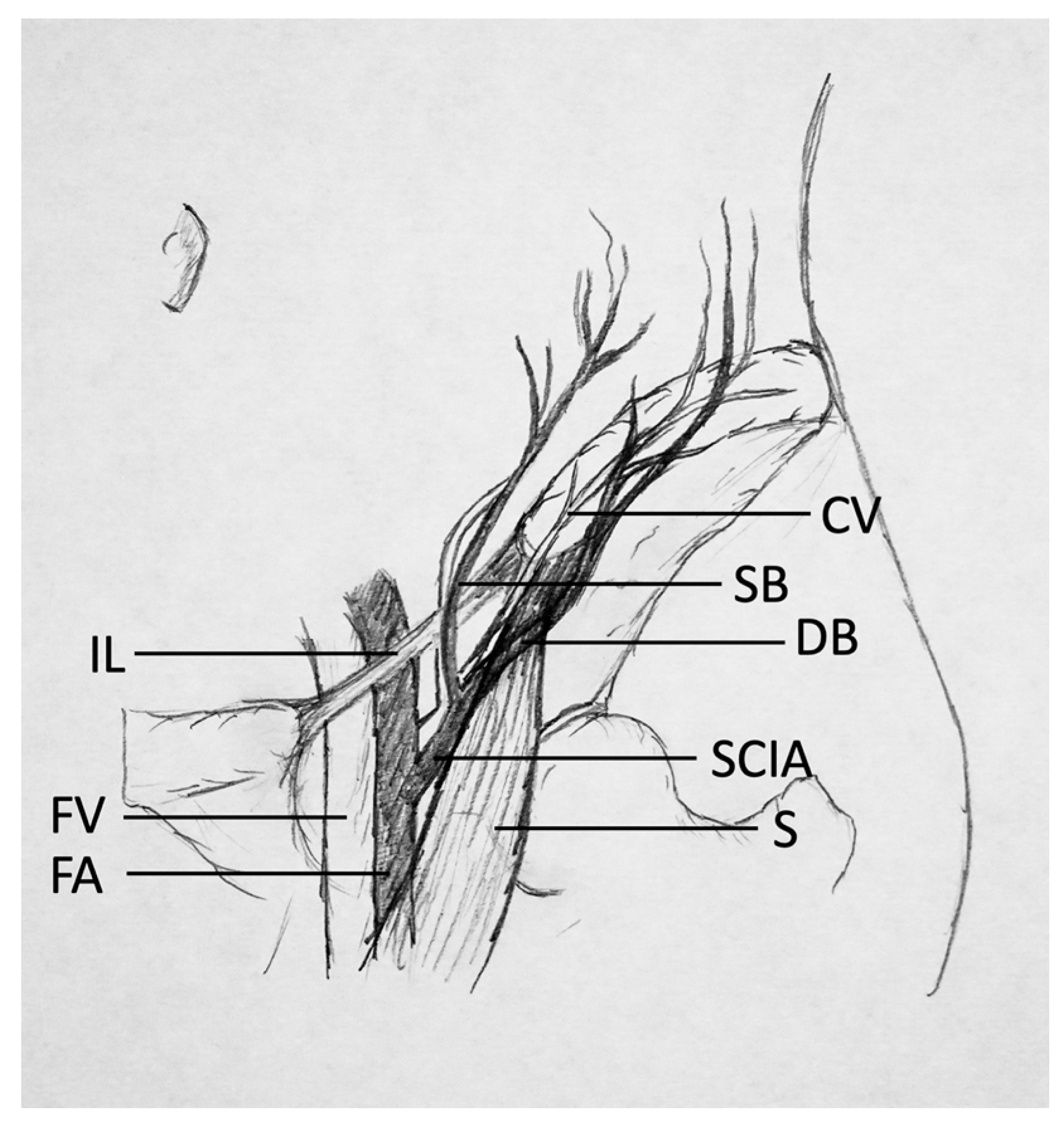The image is a detailed, hand-drawn medical diagram, likely for educational purposes, rendered in black ink or pencil on a white background. The drawing appears to depict a complex system of arteries, veins, muscles, and possibly nerves, with varying shades used to distinguish each anatomical feature—darker for arteries and veins, lighter for bones, and medium shading for muscles, which are also marked with stripes. Labeled in typewritten black letters, the diagram includes abbreviations such as IL, FV, FA on the left side, and CV, SB, DB, SCIA, and S on the right and bottom. The labeled parts are connected to their respective sections by straight, black lines, ensuring clarity in the depiction of the anatomical relationships.